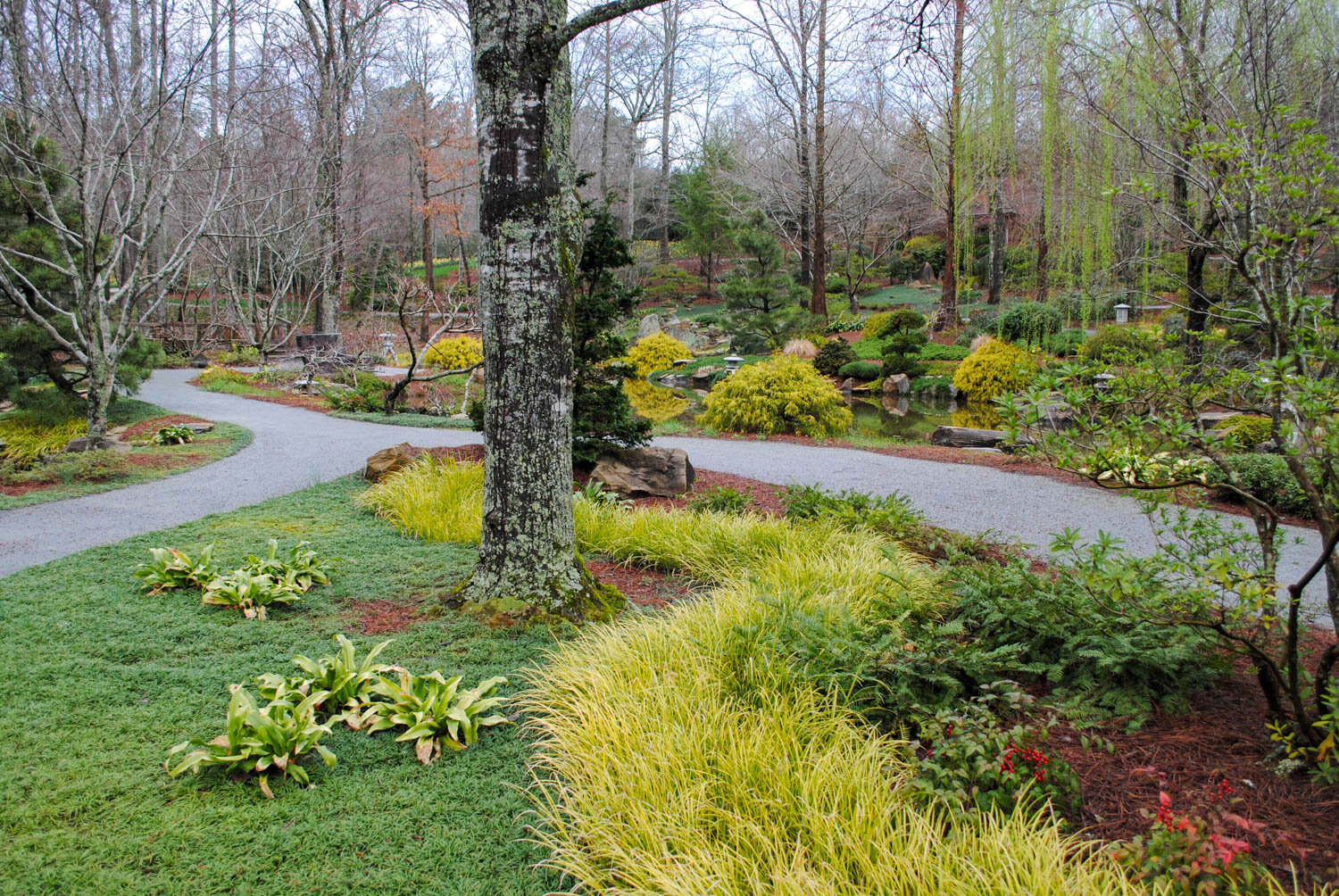The photograph depicts an outdoor setting that appears to be either a front lawn, a public park, or a professionally landscaped gardenscape. It captures a large expanse of bright green grass interspersed with a variety of trees, some bare and others showcasing sporadic red, pink, and white flowers, indicating a timeframe of mid to late winter or early spring, likely around March or early April. The sky is a light blue, almost white, providing a clear and bright atmosphere with plenty of natural light.

A concrete pathway winds throughout the scene, more likely intended for pedestrian use rather than vehicular traffic. This pathway is situated toward the right and left edges of the image, with the landscaped area full of diverse shrubs and greenery occupying the central space. Notably, some shrubs exhibit a green hue with a yellowish tint, adding to the myriad shades of green present.

In the background, there is a suggestion of a house, but it remains indistinct and partially obscured. The central focal point includes a main tree adorned with moss and white bark, adding a touch of enchantment to the scene. The overall composition is a horizontal rectangle, with professionally arranged landscaping that gracefully winds around the path, and various colors—red, brown, yellow, green, gray, black, white, and orange—offering vibrant visual interest. No text is present in the image.